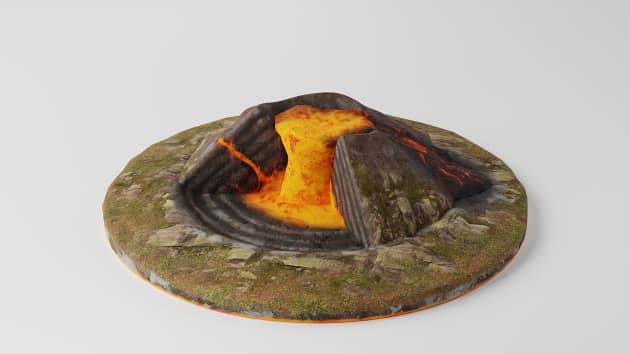This image presents a detailed, artistic representation of a scale model volcano set against a light grey or white background. The model itself, mostly occupying the foreground, effectively portrays geological features with meticulous craftsmanship, likely created using plaster or modeling clay. The volcano is embedded in a disc-shaped base, which displays realistic textures and colors—a mossy green surface interspersed with patches of brown and grey stones, suggesting vegetation and rugged terrain.

Highlighting its educational or artistic purpose, the volcano’s front section is cut away, offering a clear cross-sectional view of its inner workings. This cut-out reveals various stratified layers of brown material, simulating earth and rock layers. Dominating the core, a vivid depiction of molten lava is achieved with bright orange and reddish hues, streaking outwards, effectively illustrating the dynamic eruption process.

The overall aesthetic and structural details of both the disc and the volcano are aimed at serving as a visual exploration tool or an artistic piece, giving spectators insight into the vibrant and fiery heart of a volcanic eruption.